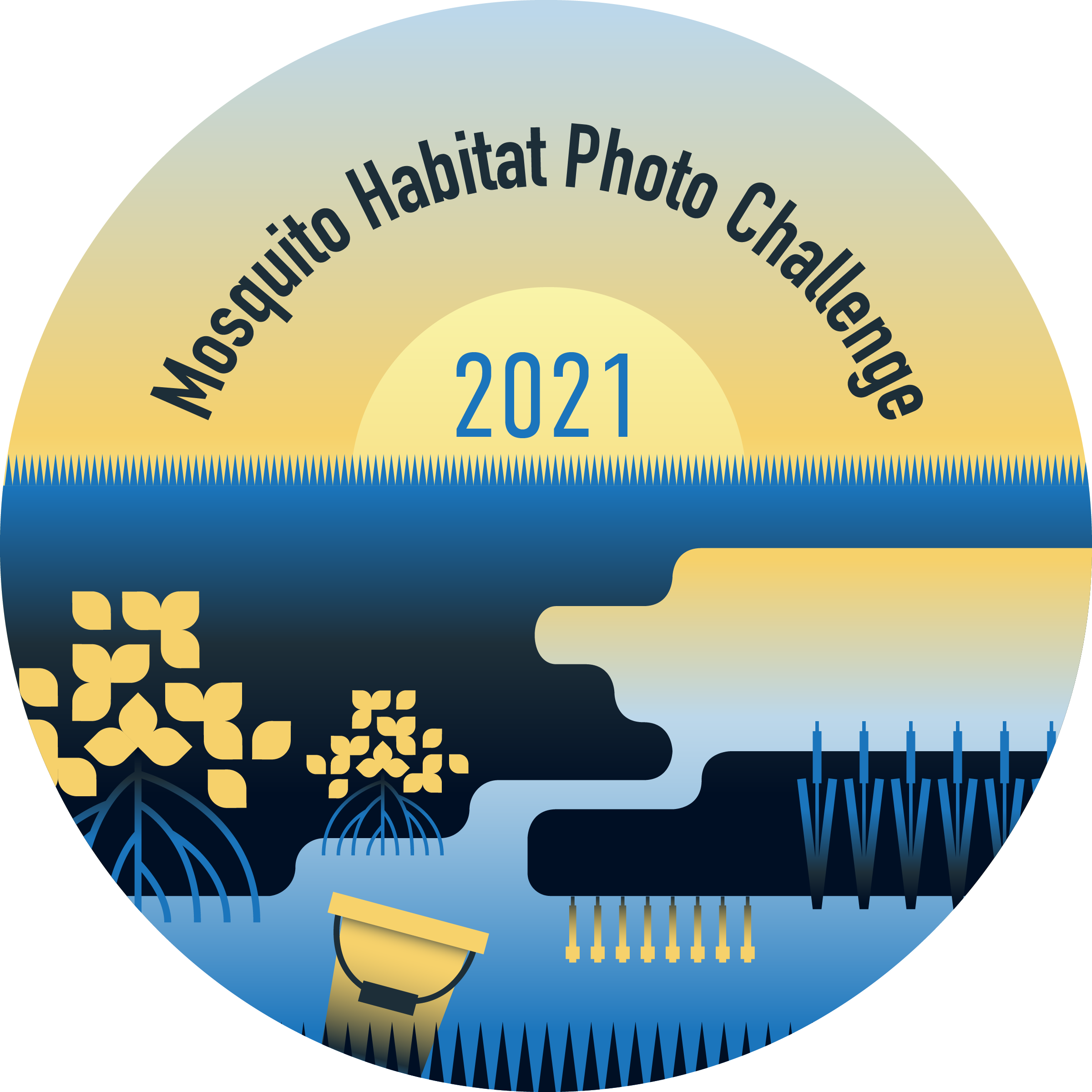The image is a circular promotional artwork for the "Mosquito Habitat Photo Challenge 2021." The design features a semicircle with the text "Mosquito Habitat Photo Challenge" displayed in black over a gradient sky transitioning from blue to orange, reminiscent of a sunset. Centered below this text is a semicircle half-sun where the year "2021" is boldly depicted in blue letters. The scene below the horizon includes a tan-colored shore leading into blue water. The foreground is populated with representations of habitats, including blue abstract illustrations of plants with visible roots, some yellow flowers, and a yellow bucket with a black handle. The composition captures a diverse natural environment, encouraging participants to explore various mosquito habitats.